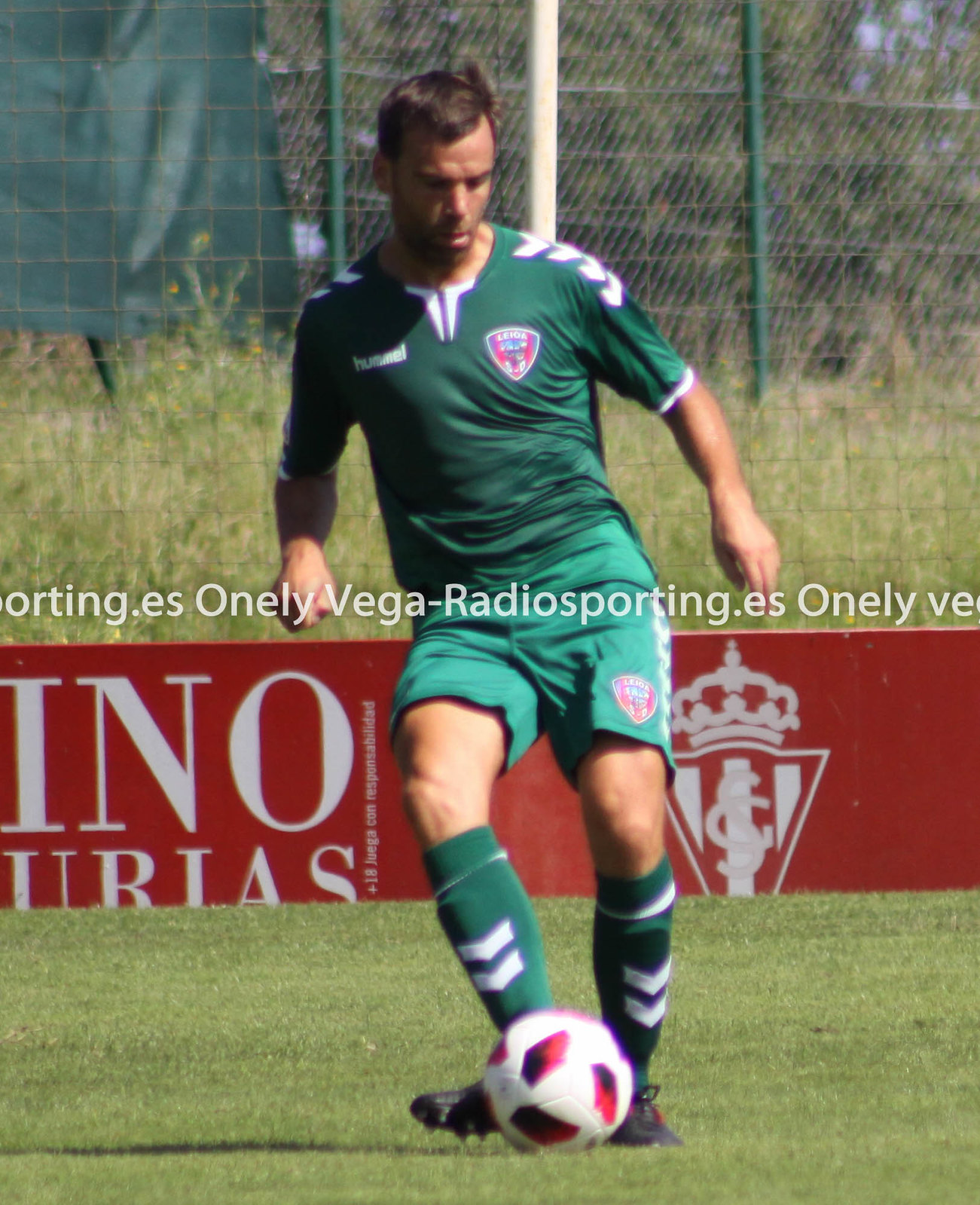In this vertically oriented outdoor photograph, a single soccer player in a green outfit dominates the scene. He wears a short sleeve green t-shirt with the brand name "Hummel" on the left chest and a badge-type logo "Lee Hoa" on the right chest, along with matching green shorts that also feature the "Lee Hoa" badge above his right knee. His green socks with white arrows reach up to his knees, and he has black cleats on his feet. His brown hair is short, and he sports a faint five o'clock shadow. The player is mid-action, looking down at a soccer ball—white with pink markings—situated near his feet, suggesting he is about to kick or dribble down the green field. A border wall in the background displays a red advertisement with white letters "sporting.es" and "onlyvega" running horizontally across the image, repeated to form the phrase "sporting.es onlyvega - radiosporting.es onlyvega." Above this wall, some netting is visible at the edge of what appears to be a stadium, with greenery in the distance. The player’s stance and focus imply he is either practicing or engaged in a game.